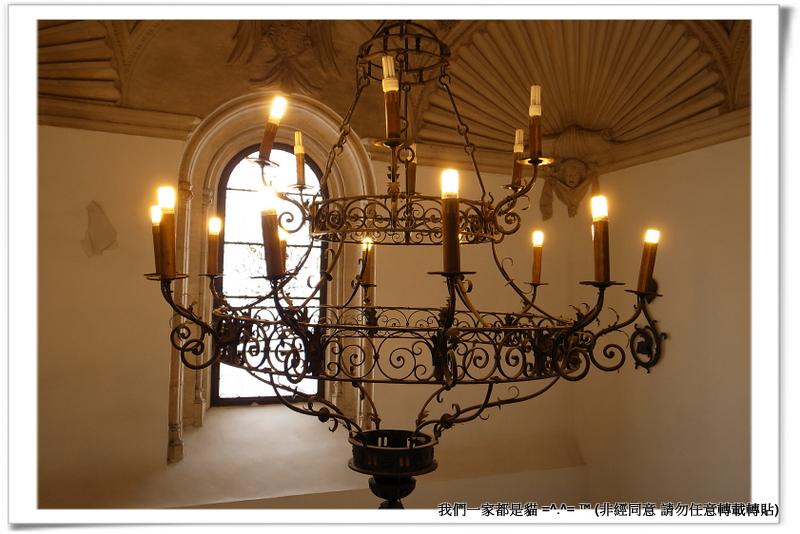This detailed photograph showcases an elegant, two-tiered chandelier crafted from a delicate iron framework or possibly a blend of bronze and copper. The chandelier features intricate scrollwork on both its primary circular tiers, with each circle supporting several sconces that resemble candelabras topped with light bulbs. The bulbs emit a warm orange hue and are slightly tilted, indicating some wear and tear. The chandelier hangs from an ornate ceiling characterized by scalloped corners, bas-relief embellishments, and a large, decorous arched window. The walls in the background appear to be either white or light yellow, contrasting with a darker, bronze or brown-toned ceiling. Additionally, there's a section of Japanese and Chinese text in the bottom right corner, set against a white-framed border.